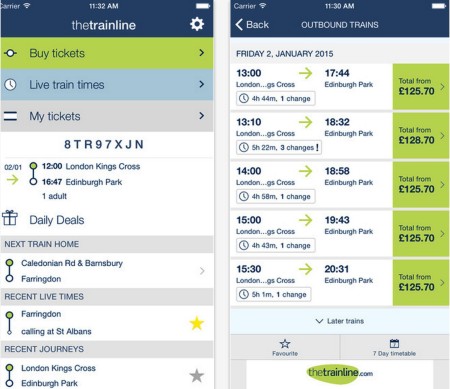The image features two screenshots of a smartphone app displaying detailed train travel information. At the top of both screenshots, the status bar indicates a carrier, Wi-Fi symbol, and the battery icon. The time displayed is 11:32 AM.

The first screenshot presents an app interface for "The Train Line" with a gear-shaped settings icon. The interface is divided into three main sections: "Buy Tickets" highlighted in lime green, "Live Train Times" in baby blue, and "My Tickets" in grey. A code "8TR97XJN" is visible, alongside a departure time of 02:01 PM and a departure station, London Kings Cross, scheduled for 12:00 PM. The expected arrival is at 04:47 PM in Edinburgh Park. It also mentions details such as "One Adult" and includes a "Daily Deals" text accompanied by a gift-wrapped box icon. Additional details show "Next Train Home" from Caledonian Road and Barnsbury to Farringdon and "Recent Live Times" from Farringdon to St. Albans—with a star indicating it is a favorite route. Additionally, it displays a recent journey from London Kings Cross to Edinburgh Park.

The second screenshot lists outbound trains scheduled for Friday, 2nd January 2015, from London Kings Cross to Edinburgh Park. The total cost for the trips is £125.70. A total of five different train options are showcased, with departure times ranging from 1:00 PM, arriving at 5:44 PM, to the latest at 3:30 PM, arriving at 8:31 PM. The background of the app is predominantly white, with green-colored text and various colored arrows indicating different data typically found in a travel app.